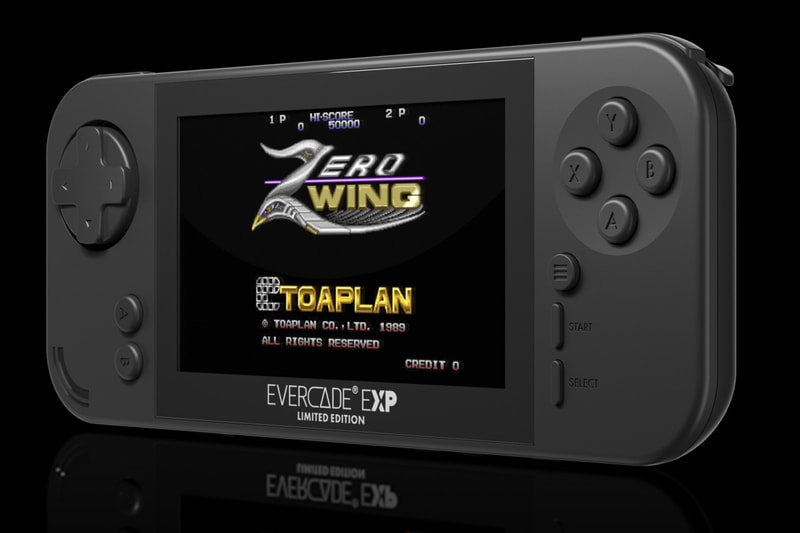The photograph showcases a handheld gaming device set against a uniformly black background. At the center of the device, there's an LED screen displaying the logo for the game "Zero Wing." The logo features "Zero" in white and "Wing" in gold, with a notably larger "Z." Above the logo, a high score of "50,000" is prominently shown, flanked by "1P" for one player on the top left and "2P" for two players on the top right. Below the logo is the text "Auto Plan," with the "O" stylized as interlocking triangles, followed by "TOA Plan" in gold. The screen also reads "Copyright TOA Plan Co Ltd 1989" and "All Rights Reserved," along with "Credit Zero."

Below the screen, the device features "Evercade EXP" in white and "Limited Edition" underneath. The device itself is light gray and rectangular. On the left side, there is a directional pad (D-pad) and two circular buttons beneath it. On the right side, there are four buttons labeled Y, B, X, and A, along with an additional circular button. Below these, two elongated buttons labeled "Start" and "Select" are visible. The matte black finish of the device blends seamlessly with the dark background, and a reflection of the gaming device is faintly visible at the bottom of the image, enhancing the overall depth and detail of the scene.